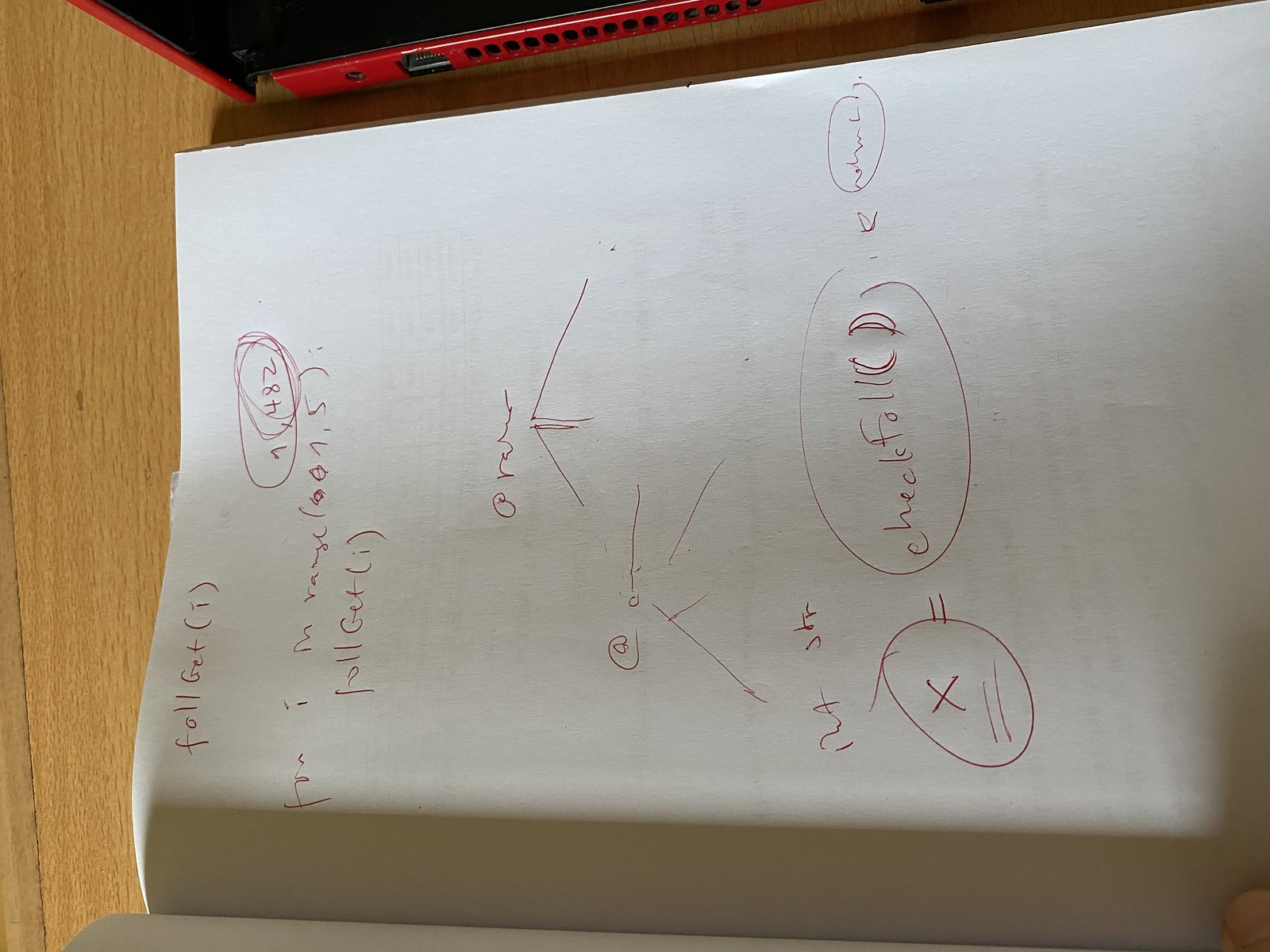In this image, a white piece of paper with handwritten notes is presented in a landscape orientation, but the writing on it is in a portrait direction, making it necessary to rotate the computer for easy reading. The writing, done with a darker red pen, includes a title at the top that reads "Fall Get (I)." The text below this initial header is largely illegible, but repeats the "Fall Get" phrase. 

Towards the right corner of the paper, the number "482" is clearly visible. The lower section of the page displays a graph featuring three converging lines meeting at a central circle, complemented by some nearby annotations. At the bottom of the paper, there is a mathematical formula with a circled "X" followed by two lines, an equal sign, and additional text which appears to be "check," "fall," and possibly another word, indicating it's some form of mathematical problem or solution, though the exact details are unclear.

The backdrop to the right of the photo comprises a wooden surface, potentially a table or floor, with a red border at its top edge and a black area above, which might be a ceiling or some molding. Adding to the scene is a red metal piece hanging from this black area, featuring a black sticker and several connecting holes, suggesting it is a component used for mounting or attachment purposes.